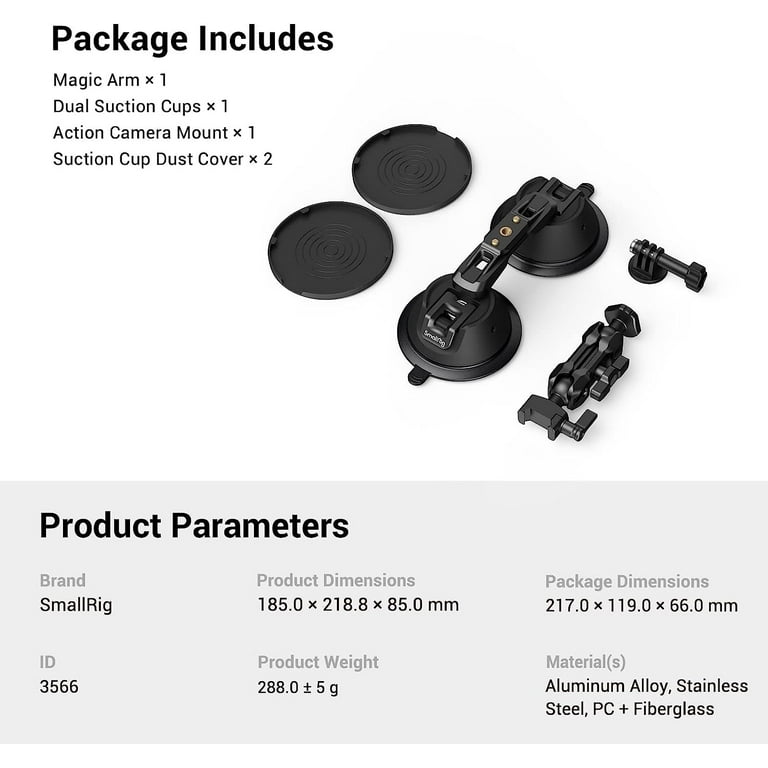This informational image, possibly from a hardware store advertisement or online catalog, showcases a product package on a clean, white background. Featured prominently are high-resolution photographs of the included components: one magic arm, one set of dual suction cups, one action camera mount, and two suction cup dust covers. Each item is black and meticulously arranged side by side, with several circular pieces and other unit shapes. The bottom section of the image presents product parameters in a gray box with black text. The brand is SmallRig, with the product ID 3566. Listed dimensions are 185x218.8x85mm, and the weight is 288 grams, with a small margin of error. Material composition includes aluminum alloy, stainless steel, PC, and fiberglass.